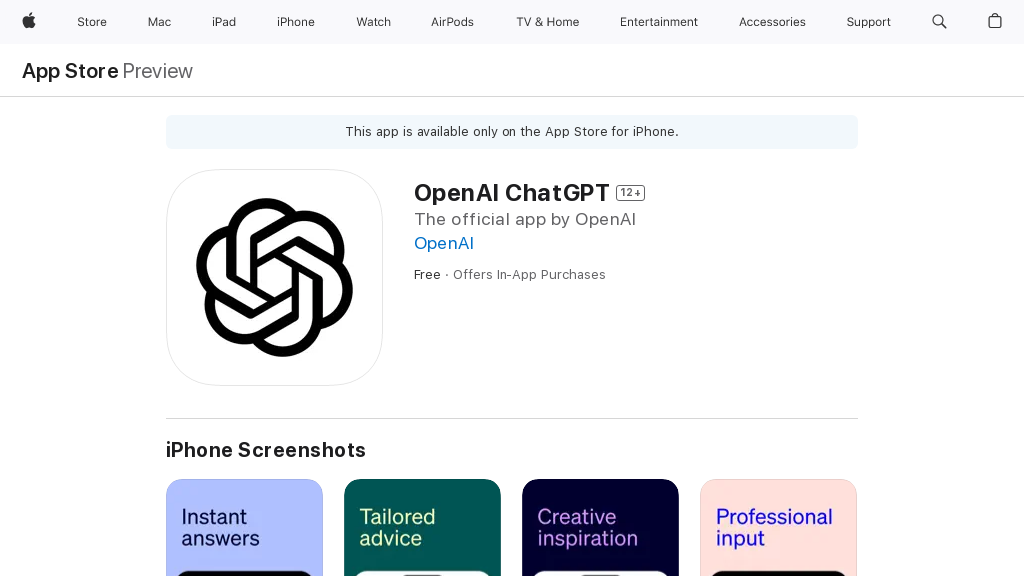**Descriptive Caption:**

This is a screenshot from the Apple Store's website showcasing the "OpenAIChatGP" app. In the top left corner, there's the iconic black Apple logo with a bite taken out of it. The header menu bar across the top is in black font and features the following categories: Store, Mac, iPad, iPhone, Watch, AirPods, TV & Home, Entertainment, Accessories, and Support. On the right side of the menu bar, there are icons for a magnifying glass (search) and a shopping bag.

Below the menu, the text "Apple Store Preview" is displayed, with "Apple Store" in a bold dark font and "Preview" in a lighter font. A light gray horizontal divider line separates this from the description below.

The text underneath states, "This app is available only on the App Store for iPhone." In a darker font, it mentions "OpenAIChatGP 12+," followed by "The official app by OpenAI" with a clickable blue link for OpenAI. The app is labeled as "Free" and mentions it "Offers in-app purchases." 

To the left of this text, there is a circular logo featuring intertwined chains in a dark black color. 

Toward the bottom of the screenshot, "iPhone Screenshots" is noted, followed by another menu listing features such as Instant Answers, Tailored Advice, Creative Inspiration, and Professional Input. The overall layout is symmetrical and well-organized, creating a clean and straightforward representation of the webpage.